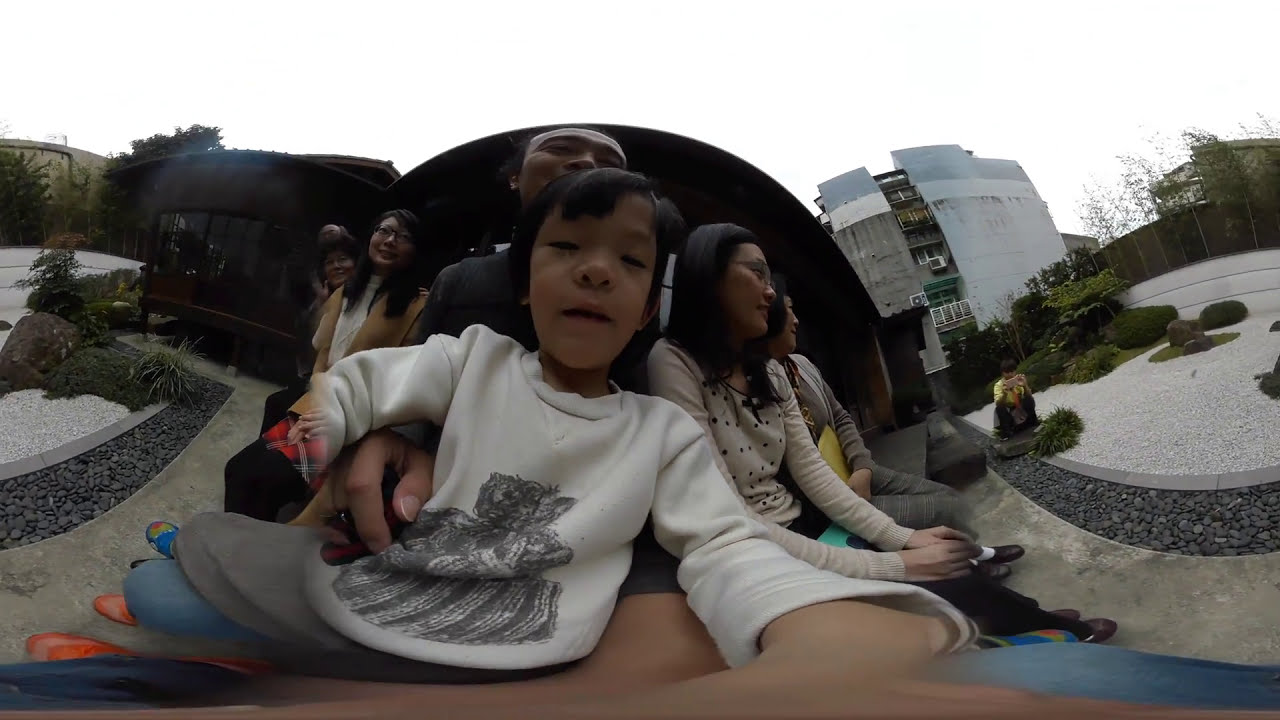In this peculiar and distorted image, a small girl wearing a long-sleeved white sweater with gray imagery on the front appears to be the primary focus. She is either sitting in the lap of or very close to a man behind her, who is dressed in a black shirt. The young girl, possibly taking the photo herself using a VR or 360-degree camera, has short hair and holds the device, resulting in the warped appearance of their surroundings.

Surrounding them is a group that seems to consist of family or friends. To the girl's right, a woman wearing a beige shirt with dots and dark pants is seated, while to her left, another woman in a tan blazer over a white shirt can be seen. Positioned on some concrete benches, the group sits amidst a setting featuring buildings, greenery, and trees. One of the buildings is multi-storied and white and gray in color, while nearby, a sidewalk leads toward another structure. The background includes rock areas and what looks like a small botanical garden.